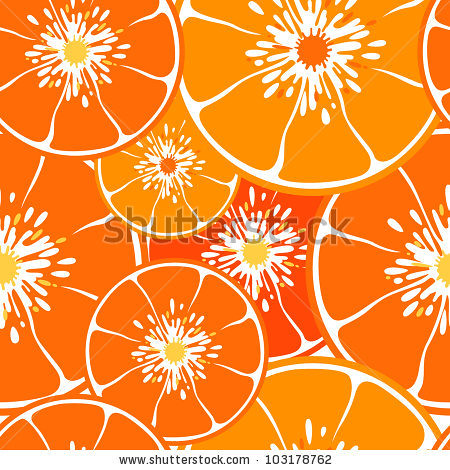This digital image features an artistic depiction of variously colored orange slices arranged in a pattern. Displayed with a watermark across the center that reads "Shutterstock," the image includes a detailed assortment of slices showcasing hues from light orange to deep blood orange. Each slice is intricately illustrated to highlight the pith and wedges, with the white inner layer and the darker orange peel surrounding them. The centers of the slices vary in color from yellow to darker orange and red, adding vibrancy to the predominantly orange composition. At the very bottom of the image, in dark grey text, is the Shutterstock website "www.shutterstock.com" along with an identification number "103178762," indicating that this might be a stock image designed for use as a desktop wallpaper or background. The interplay of different shades and accents creates a vivid and detailed visual.